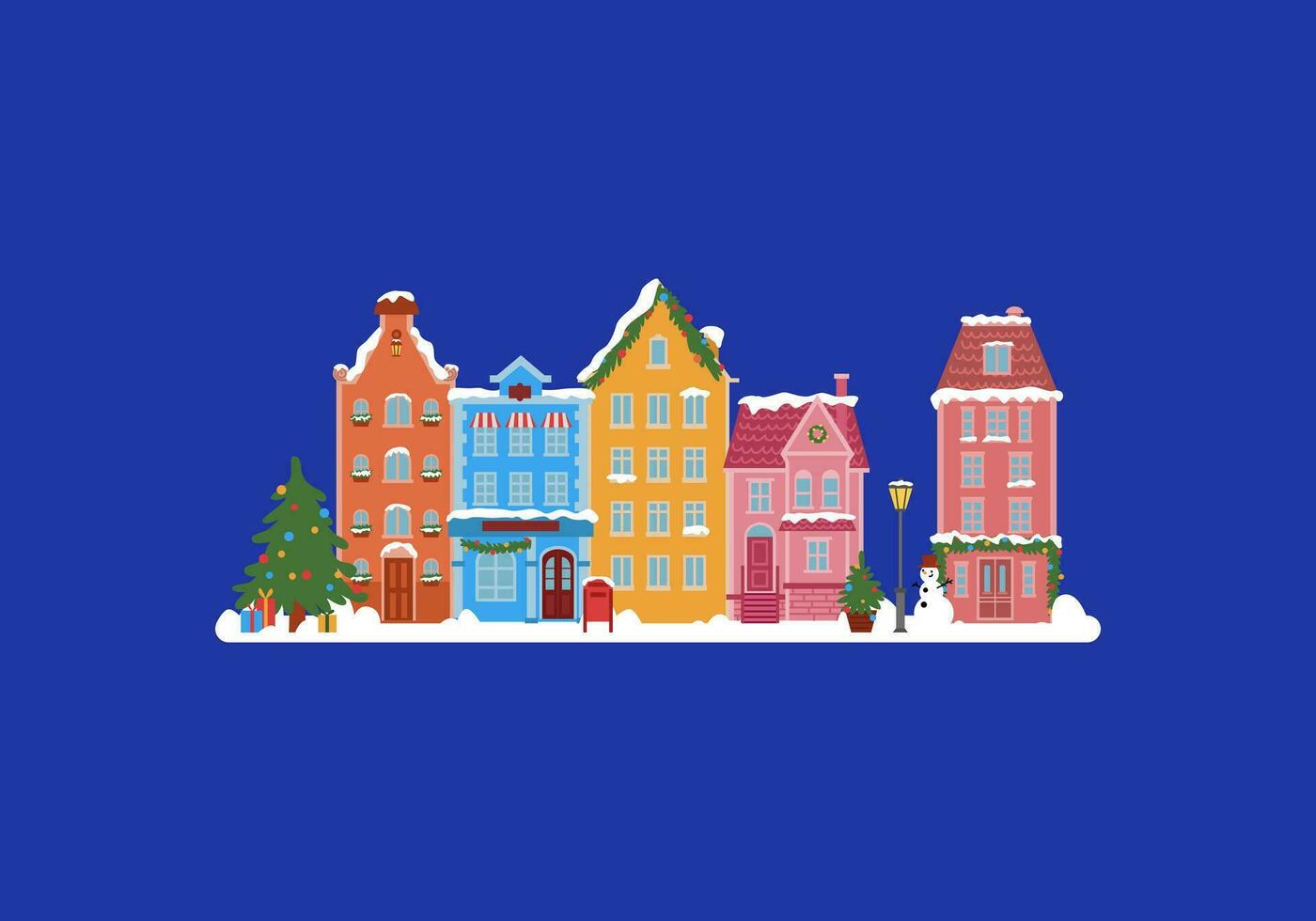In this animated image, a festive winter scene is depicted with a row of five houses set against a blue background. To the far left, a vibrant green Christmas tree adorned with red, yellow, and blue ornaments stands tall with three presents at its foot. Directly beside the tree is an orange building, the second tallest in the scene, featuring tiny windows and a larger door in a darker shade of orange.

Adjacent to this, a blue house with six first-floor windows and a single large window on the ground floor is framed by a brown door with glass. Following this is a yellow building decorated with Christmas tree leaves and matching ornaments on its roof, and thirteen windows that give it a festive look.

Next in line is a pink-colored house with a darker roof and door, featuring four windows and a small potted Christmas tree displaying similar ornaments. A black, lit lamppost stands between this house and a smiling snowman adorned with a brown hat. 

On the right-most side, a reddish-pink house with seven windows on the upper floor and two on the lower floor is embellished with Christmas tree leaves and ornaments at the ground level. Snow covers the rooftops and ground, adding to the holiday atmosphere.